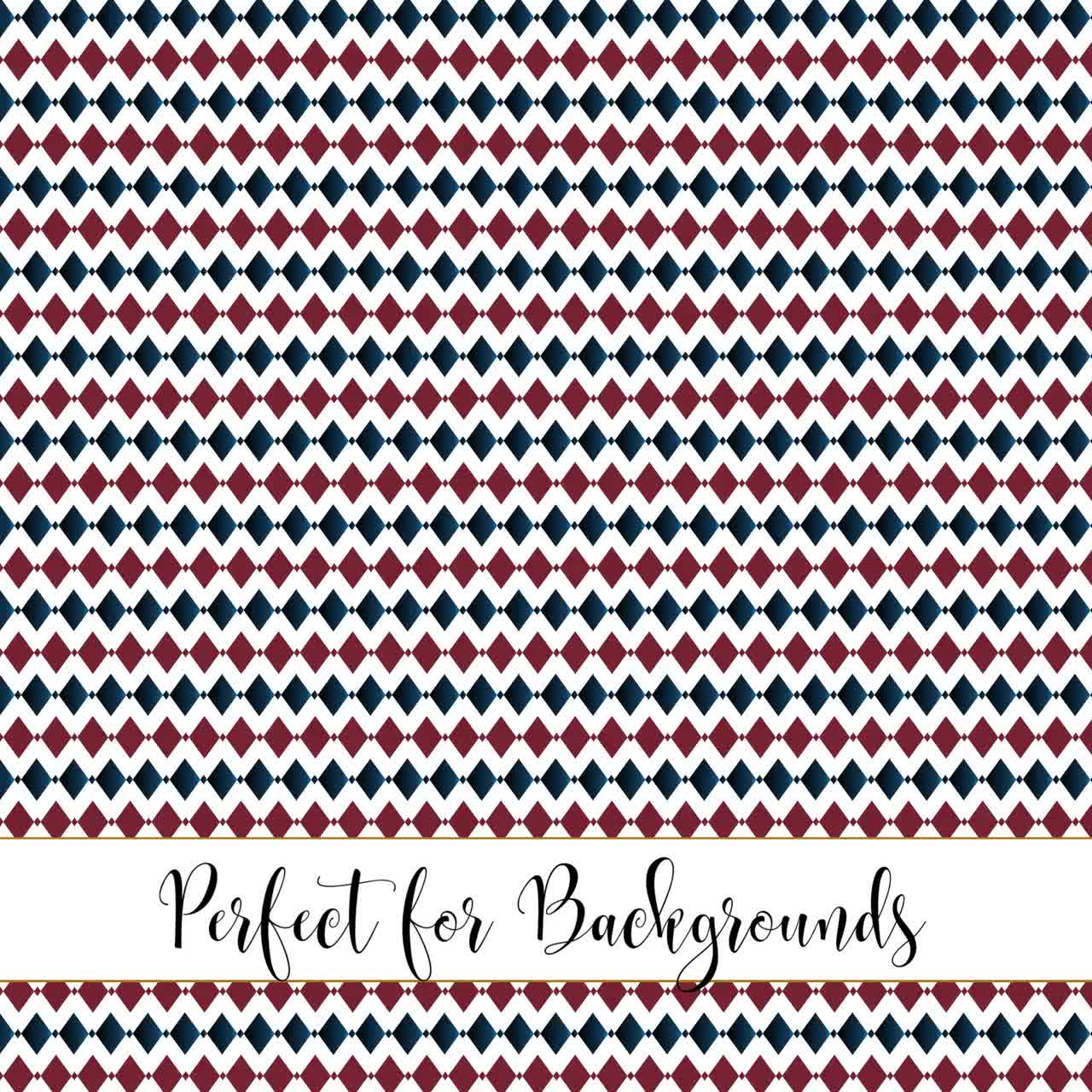This computer-generated image is designed as a background, featuring a mesmerizing diamond pattern with rows of interconnected small diamond shapes. The alternating rows showcase two main colors: maroon (or burgundy) and black, creating a visually striking and repetitive pattern. Situated just above the bottom three rows, the phrase "Perfect for backgrounds" is displayed in a black script font against a white backdrop, subtly accented by gold borders above and below the text. The entire composition, devoid of any additional imagery or borders, presents a clean and captivating design intended for use as a background.